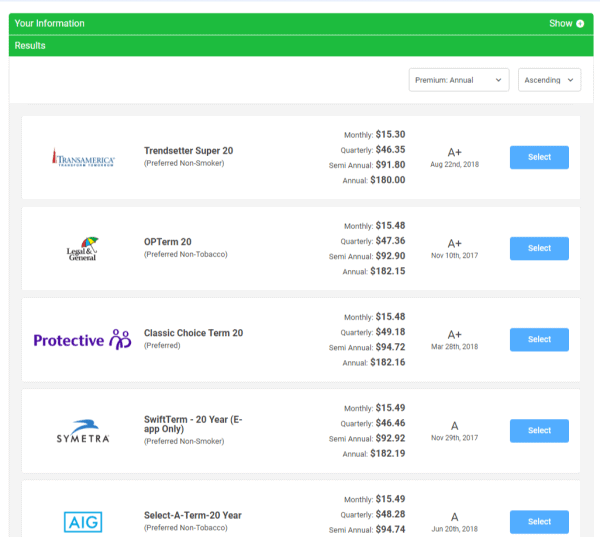Screenshot of an Insurance Quote Portal

This image is a detailed screenshot of an insurance quote portal. At the top, the page header reads "Your Information," followed by buttons labeled "Show" and "Results" at the bottom. Users can filter the insurance plans by premium options—such as monthly, quarterly, semi-annually, and annually—and organize the results in ascending order.

Displayed are several insurance plans from different providers, including Transamerica, Legal & General, Protective, Symmetra, and AIG. Each plan has a preferred non-smoker or non-tobacco classification and is accompanied by a select button. Below are the specifics of each plan:

1. **Transamerica Trendsetter Super 20**
   - Preferred Non-Smoker
   - Monthly: $15.30
   - Quarterly: $46.35
   - Semi-Annual: $91.80
   - Annual: $180.00
   - Rating: A+ (August 22, 2018)

2. **Legal & General OP Term 20**
   - Preferred Non-Tobacco
   - Monthly: $15.48
   - Quarterly: $47.36
   - Semi-Annual: $92.90
   - Annual: $182.15
   - Rating: A+ (November 10, 2017)

3. **Protective Classic Choice Term 20**
   - Preferred
   - Monthly: $15.48
   - Quarterly: $49.18
   - Semi-Annual: $94.72
   - Annual: $182.16
   - Rating: A+ (March 28, 2018)

4. **Symmetra Swift Term 20-Year E-App Only**
   - Preferred Non-Smoker
   - Monthly: $15.49
   - Quarterly: $46.46
   - Semi-Annual: $92.92
   - Annual: $182.19
   - Rating: A (November 29, 2017)

5. **AIG Select-a-Term 20-Year**
   - Preferred Non-Tobacco
   - Monthly: $15.49
   - Quarterly: $48.28
   - Semi-Annual: $94.74
   - Annual: Data Cut-Off
   - Rating: A (June 20, 2018)

This snapshot concisely presents the available insurance options, allowing for easy comparison of premium costs and provider ratings.